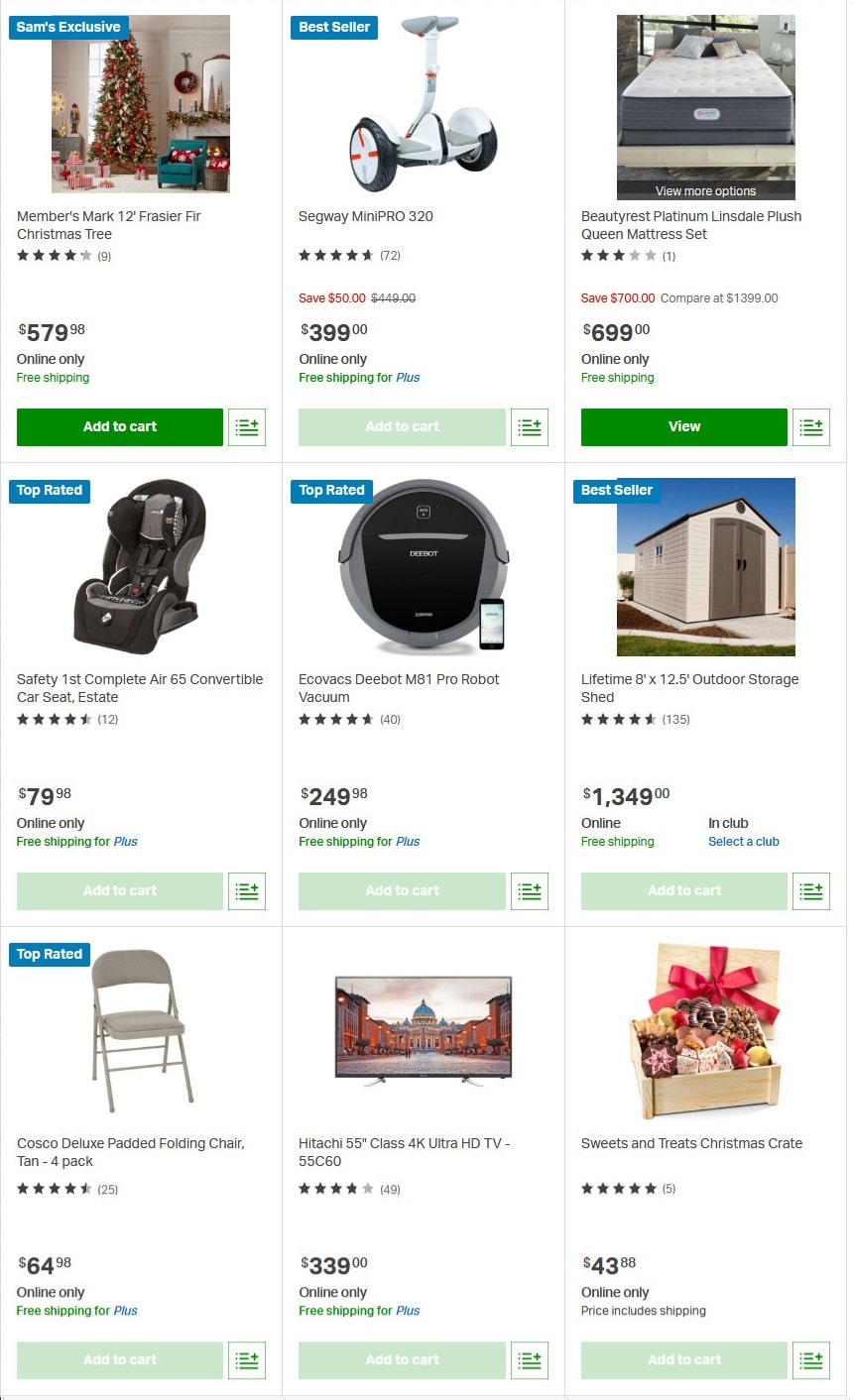This vertical image appears to be a section from an online retail webpage, reminiscent of an Amazon-like shopping platform. The layout features three rows, each displaying three products side by side in vertical rectangular frames.

- **First Row:**
  1. **Upper Left Corner:** A turquoise box with white text reads "Sam's Exclusive." Below it, an image showcases a family home decorated with a Christmas tree. The item is identified as "Member's Mark," garnering 4.5 stars and priced at $579.96. A green "Add to Cart" button is visible at the bottom.
  2. **Center:** Labeled "Best Seller," the product is a Segway scooter priced at $399, though the specific text is somewhat blurry. The "Add to Cart" button for this item is grayed out.
  3. **Right:** Displaying a set of mattresses priced at $699, this product features a green "View" button at the bottom.

- **Second Row:**
    1. **Left:** A car seat labeled "Safety First Complete," adorned with a "Top Rated" blue rectangle. The price is $79 and some cents. The text below mentions "Online Only" and offers "Free Shipping" in green font, though specifics are hard to read. The "Add to Cart" button is grayed out.
    2. **Center:** Another "Top Rated" product, though the image and details are unclear.
    3. **Right:** Featuring an outdoor storage shed labeled "Best Seller." It comes with a free shipping offer highlighted in green. The corresponding "Add to Cart" button is grayed out.

- **Third Row:**
    - This row continues the pattern established in the first two rows, with product details that are similarly structured but too indistinct to describe precisely.

Each product image also contains the item's name, star rating, price, and a purchase button, either "Add to Cart" or "View," indicating user access options. The black font used for item descriptions and prices varies in legibility, and the presence of grayed-out purchase buttons suggests some products are unavailable for immediate online purchase.